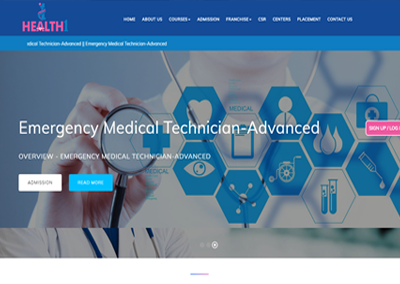The image showcases a web page with distinct elements organized in a structured layout. At the top of the page, there is a prominent blue navigation bar. On the left-hand side of this bar, "Health" is displayed in pink, accompanied by a small, indistinct logo above it. To the right of the "Health" logo, several navigation links are visible in white text, reading "Home," "About Us," an unclear item, "Admissions," followed by sequential numbers "1, 2, 3, 4, 5," and concluding with "Contact Us."

Beneath this primary blue bar, there is a lighter blue bar also containing some text in white, although the specific wording is unreadable. The main content below these bars features a background photograph of a person's hand holding a magnifying glass. The person, sporting a white coat, is shown from the chin down to about the chest. Superimposed onto this image are various shapes and medical-themed graphics.

In large, white text across the photo, the words "Emergency Medical Technician - Advanced" are displayed. Offset to the right of this text is a pink button with unreadable white text. Below the main photograph, the caption "Overview Emergency Medical Technician Advanced" is displayed, accompanied by two buttons. One button, labeled "Admission," is white, while a second, unreadable button is blue.